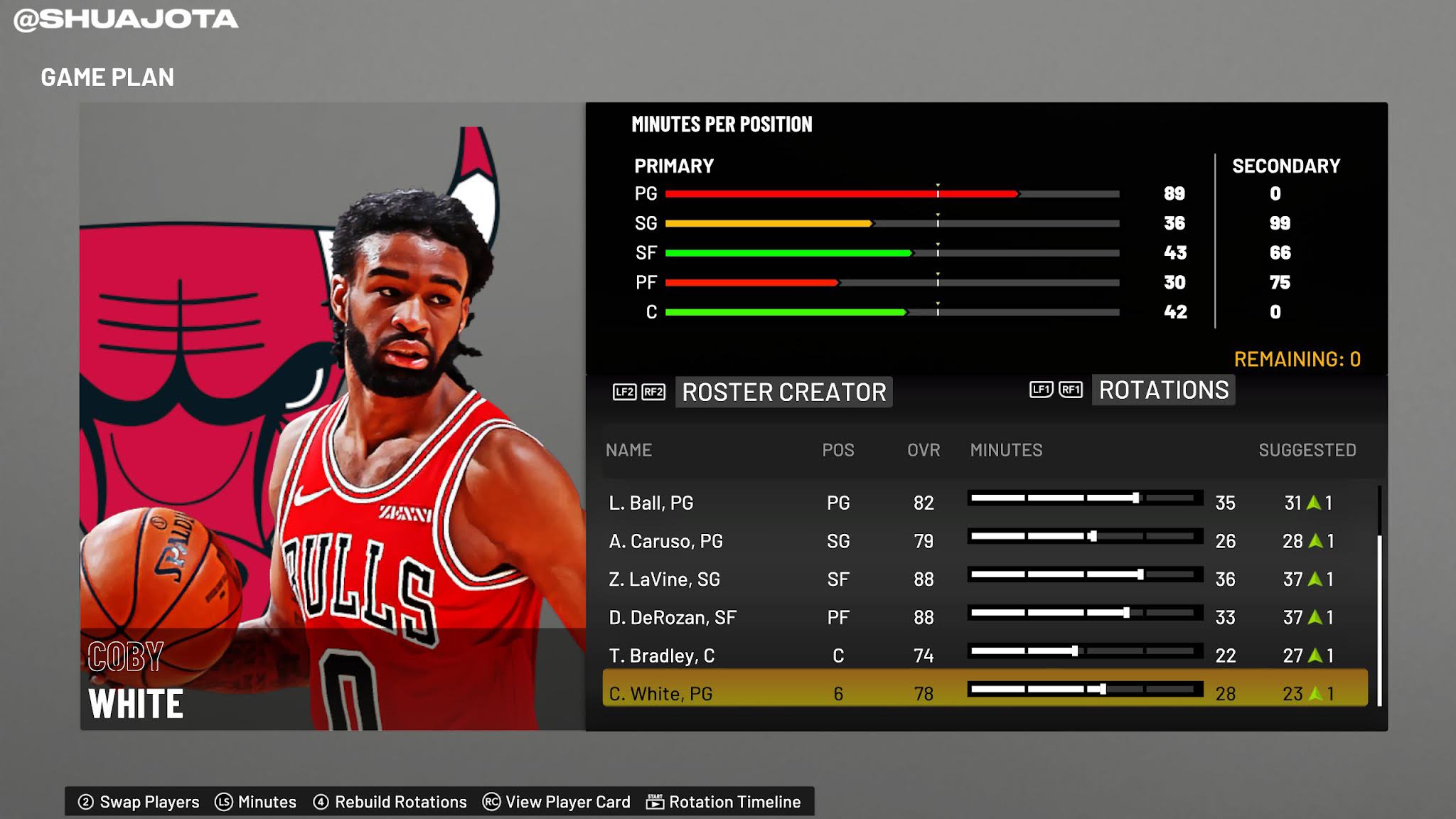This image is a screenshot of a sports website, identified as "SHUAJOTA" in bold white font located in the top left corner. Directly beneath this title, it reads "Game Plan." 

The central feature of the image is a square box displaying the Chicago Bulls logo set against a background featuring a Chicago Bulls basketball player. The player, an African-American male with dreadlocks and a beard, is holding a basketball in his right hand. The text "Kobe White" is positioned at the bottom left corner of this image, identifying the player.

To the right of this image is a section titled "Minutes Per Position" against an entirely black background. This section presents data in a series of colored lines indicating the player's usage by position:
- PG (Primary) is marked by a red line reaching up to 89
- SG (Secondary) is marked by a yellow line reaching up to 36
- SF (Small Forward) is marked by a green line reaching 43
- PF (Power Forward) is marked by a line reaching 30
- C (Center) is marked by a green line reaching 42

Below this section, it reads "Roster Creator" accompanied by additional information and boxes. On the far right of the image is a section titled "Rotations," which includes two boxes filled with data. In the upper right corner of this section, it states "Secondary," with figures 0, 99, 66, 75, and 0 listed beneath it.

At the bottom left of the image, there is text listing various player names along with their positions and statistics, including "PDS," "OFR," and suggested minutes. Highlighted at the bottom is "C. White, PJ, PG." The entire layout is designed to provide a detailed overview of the game plan and player statistics for the Chicago Bulls, with a focus on Kobe White.